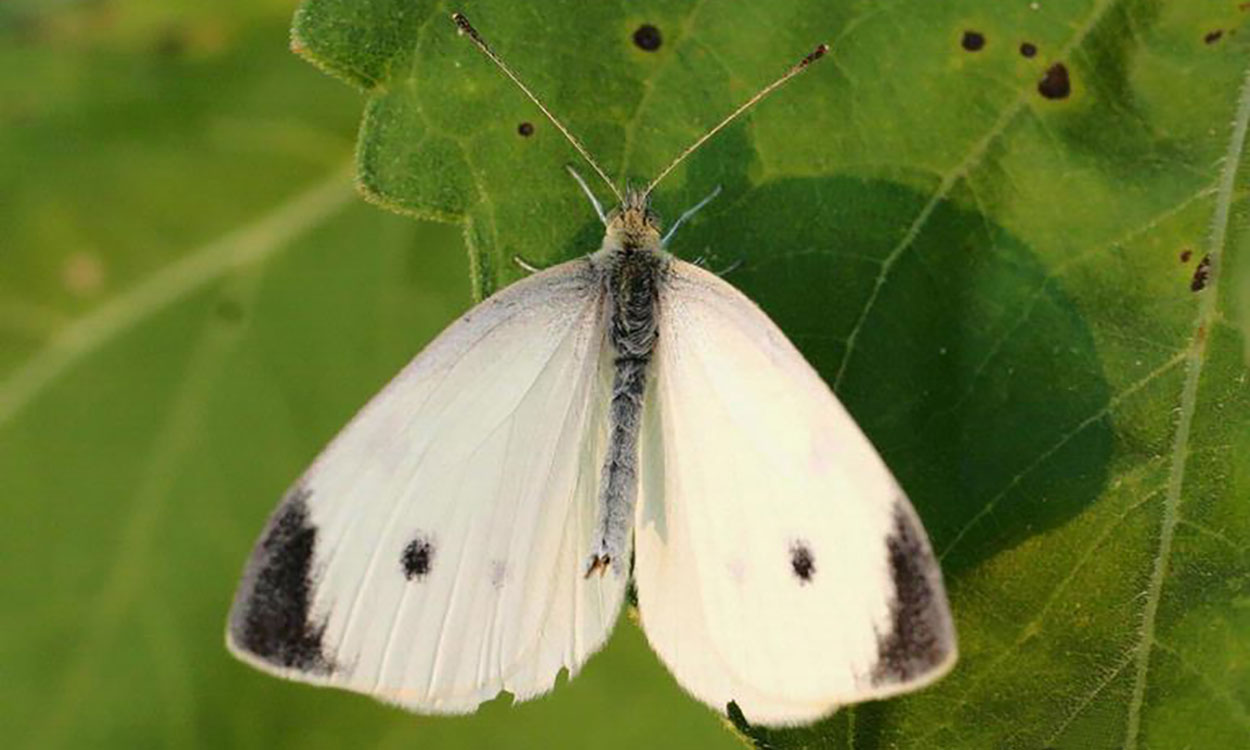The detailed photograph captures a striking up-close view of a white moth positioned on a bright green leaf. The image is in a landscape orientation, longer than it is tall. The focal point is the moth, which takes up around 25-30% of the image, situated toward the lower edge and centered horizontally. The moth, facing upward with its yellow head and two prominent long antennae at the top, features a body that is gray and fuzzy. Its large symmetrical wings are a predominant white, adorned with one small black polka dot in the center of each wing, and black or dark gray tips. The vibrant green leaf, larger than the moth and marked with some black splotches, forms the immediate backdrop. Beyond, the blurred background reveals additional leaves, subtly hinting at a lush, green environment.